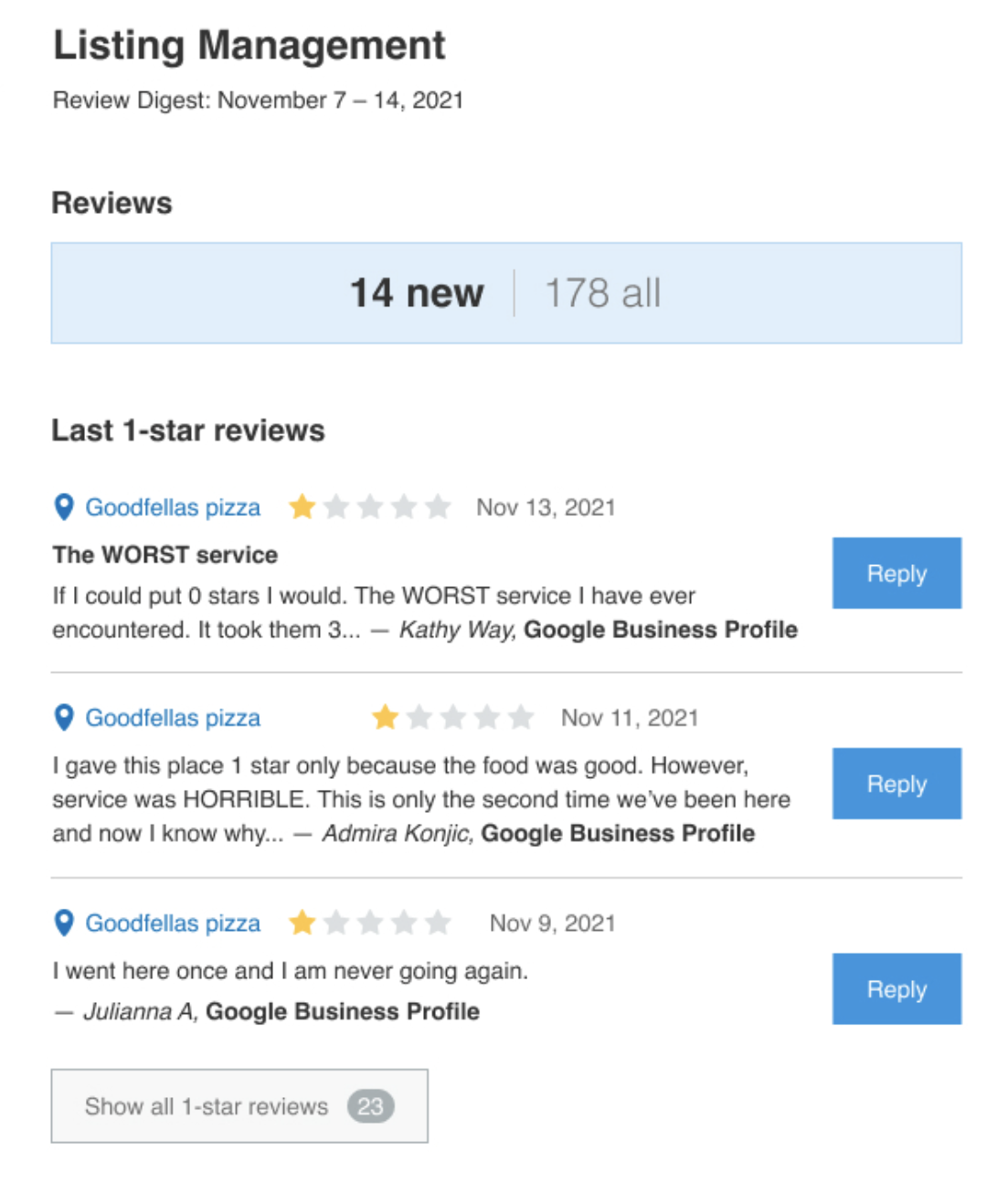This image is a detailed screenshot from the "Listing Management - Review Digest" for the period of November 7th to 14th, 2021. The digest highlights 14 new reviews, with a cumulative impact of $178. Among these, it prominently features a series of one-star reviews, indicating significant customer dissatisfaction with Goodfellas Pizza.

In bold, a particularly scathing review reads: "The worst service. If I could give zero stars, I would. The worst service I have ever encountered." This review, posted on November 11th, 2021, trails off with a cryptic mention of "three Kathewathys."

Another reviewer, Admiriak Konadjic, left a one-star review on November 13th, 2021, stating, "I gave this place one star only because the food is good. However, the service was horrible. This is only the second time I've been here and now I know why."

Additionally, Julian A., another disgruntled customer, declared, "Went here once and I’m never going here again," contributing to the growing collection of one-star reviews.

Overall, the image underscores Goodfellas Pizza's struggle with customer service, as evidenced by the option to view all 23 one-star reviews and the array of blue reply buttons alongside each mini-review. It appears on a platform reminiscent of a review aggregation site, similar to Yelp or the Better Business Bureau, where businesses can manage and respond to their customer feedback.